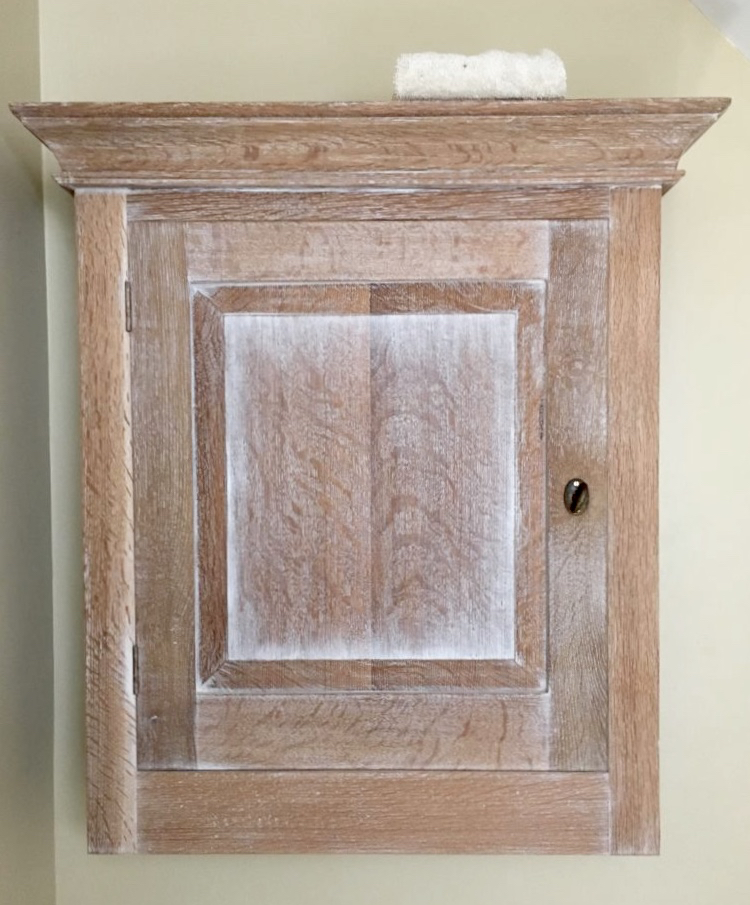The photograph depicts a wooden wall-mounted cabinet with a distinct rectangular shape, slightly wider at the top, resembling a classical design often seen in medicine cabinets. The cabinet is affixed to a light-colored wall, which appears to be a pale green or an off-white hue, positioned in a corner where the adjacent wall shares a similar light shade. The top of the cabinet features a flared, flat surface that functions as a shelf, where a neatly folded white terry cloth towel is placed. The cabinet door, secured with a lock on the right side, is equipped with an oval-shaped dark bronze knob opposite the hinges. Decorative yet functional, the cabinet's harmonious design elements and the minimalistic color palette, emphasizing the wood tones and white accents, make it the focal point of the image, suggesting its potential relevance for a design or woodworking showcase.